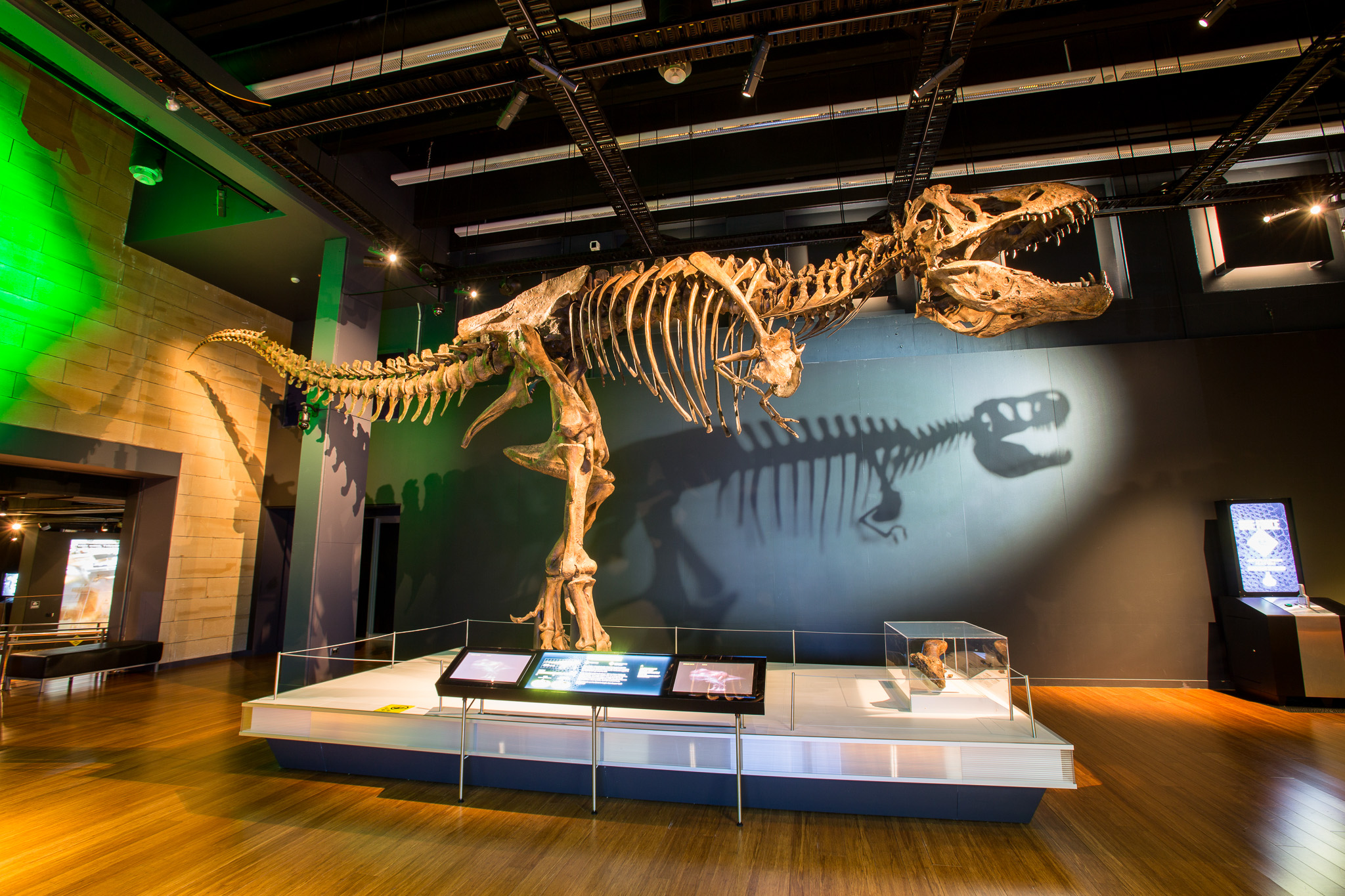In this detailed photo, a prominent T-Rex skeleton, characterized by its striking orangish-brown bones, stands majestically on a glossy white rectangular display base within a museum setting. The gleaming wooden flooring highlights the pristine presentation of the exhibit. Facing to the right, the T-Rex casts a dramatic black shadow on the gray wall behind it, illuminated by a spotlight that accentuates the intricate details of the fossil. 

In the foreground, three informational display plaques are positioned in front of the base, providing additional context about the T-Rex. To the left of the image, a vivid neon green light draws attention, while to the right, a glowing interactive kiosk invites engagement. The museum's ambiance is complemented by a black and silver roof structure, with white encased lights casting a bright glow. A yellow brick wall featuring a black-framed doorway and additional black posts are visible in the adjacent room. 

The display is encased by clear glass from waist height down, safeguarding some smaller bones displayed within a separate glass case beneath the T-Rex. Reflective surfaces enhance the clean, sophisticated atmosphere, further emphasized by the ceiling's catwalks and meticulously maintained environment.